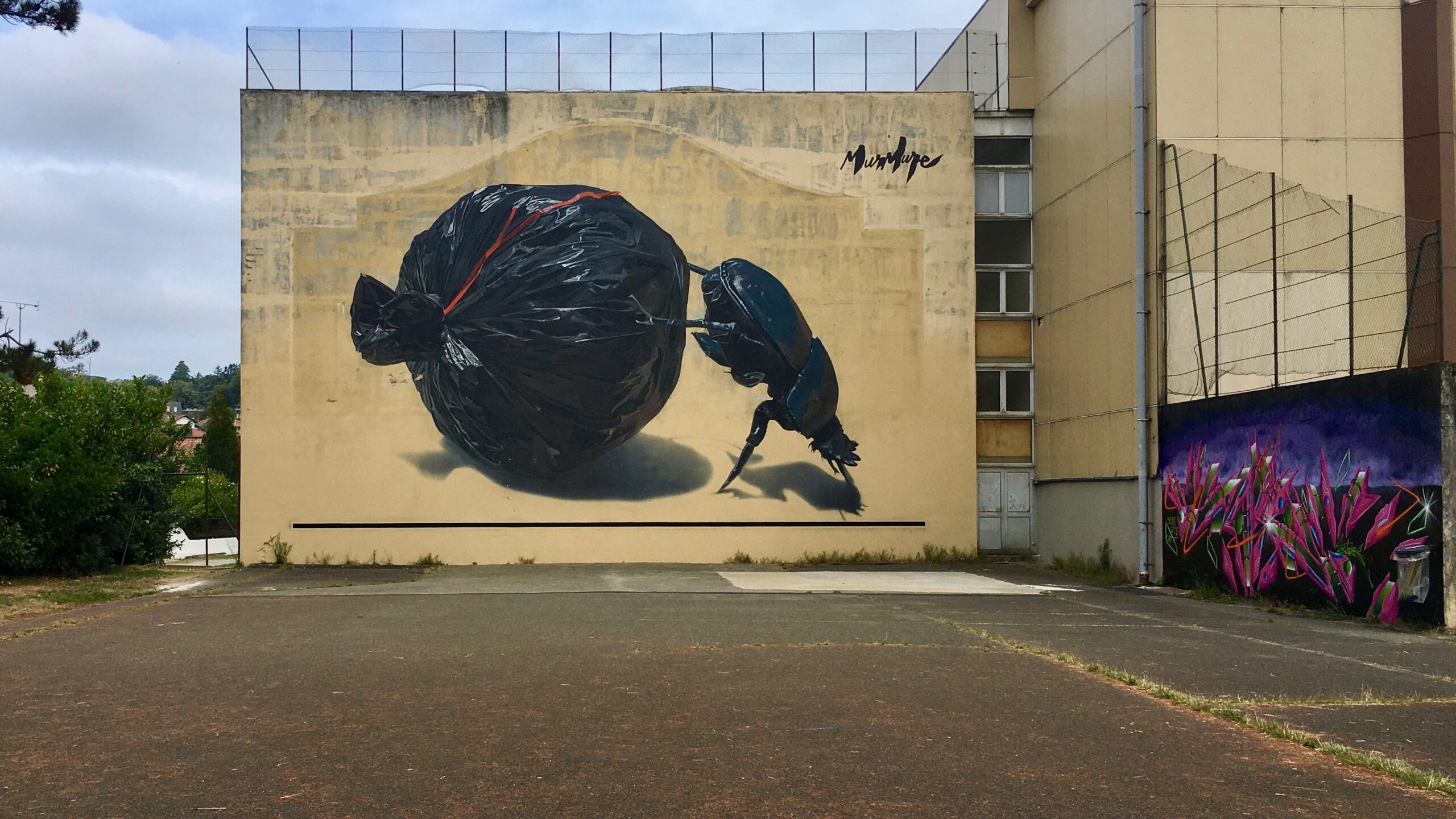This daylight photograph captures an outdoor scene featuring a large mural on the wall of an older, tan building. The mural is a realistic and amusing depiction of a glossy black dung beetle rolling a trash bag with a red tie, instead of the usual dung ball. Shadows cast to the right add depth to the mural. The image showcases part of the side and back of the four-story building, revealing a slightly dirty yellow façade with minor signs of weathering.

In the foreground, there is an empty concrete parking lot leading to the building. To the left of the mural, there are lush green bushes and trees. On another wall to the right, a vibrant pink and purple abstract sculpture-like painting adds more artistic flair to the scene. There are a few windows visible on the far right of the building, and a wire fence extends from the building to the right, supported by long poles. The artist's signature, which starts with an "M," is located in the top right corner of the mural. The sky and clouds can be seen peeking through the background, completing the outdoor setting.